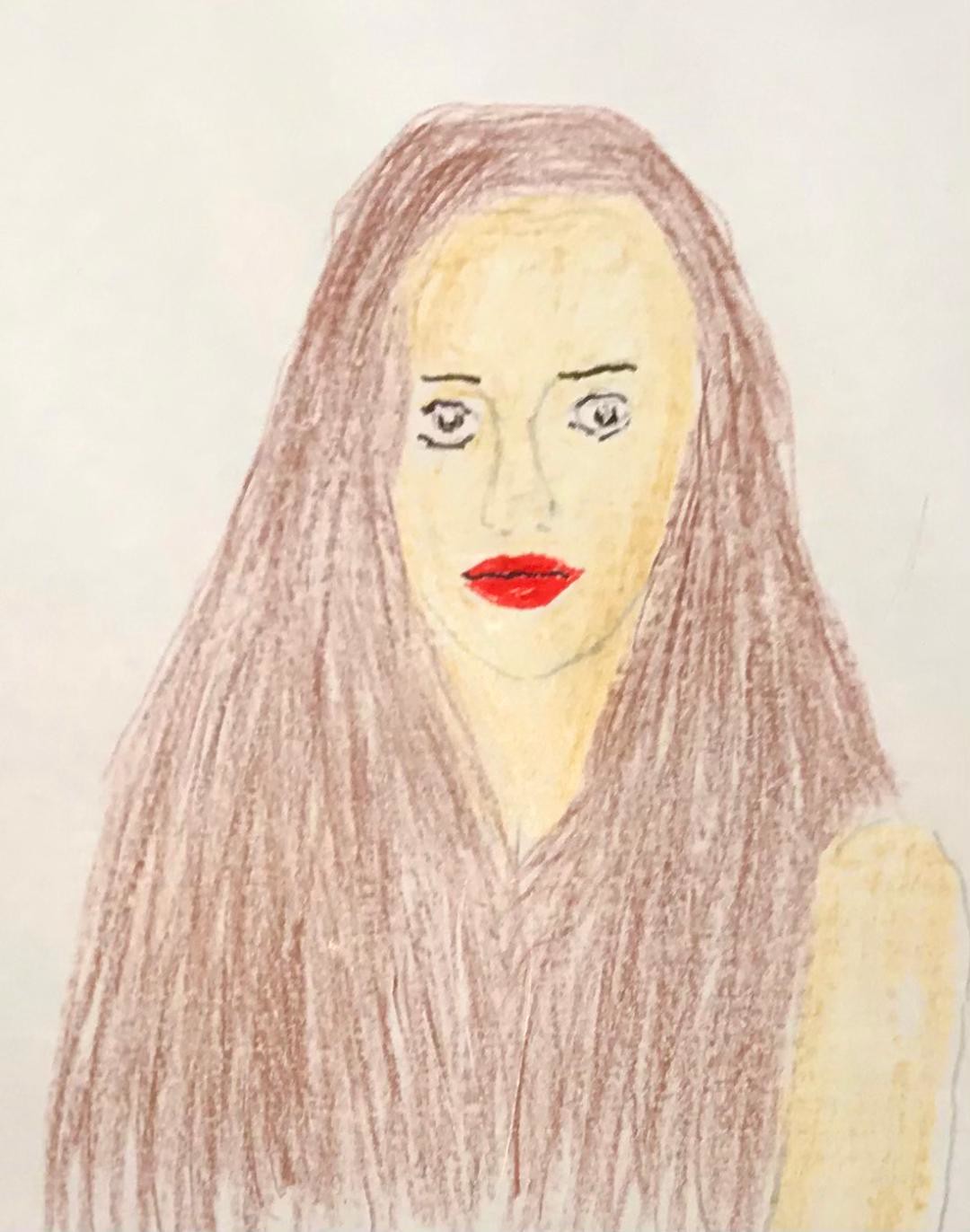This detailed colored pencil drawing depicts a woman with striking features. She has voluminous, chestnut brown hair that cascades down over her chest, completely covering it. Her right shoulder is exposed, while her left shoulder remains concealed beneath her flowing hair. Her lips are vividly colored red, with a black squiggly line in between to enhance definition. Her eyes are wide, with vertical line eyebrows that add to her expressive gaze. Her hair is parted to the left and meticulously shaded in brown, lending a sense of depth and texture.

The artist has used a yellow colored pencil to color her face and arm, creating a warm and luminous effect. Her nose, sketched in pencil, features a unique design where it bows in the middle, angling upward from the left nostril to the center and then curving back down at the other nostril. This distinctive style contributes to the overall uniqueness of the portrait.